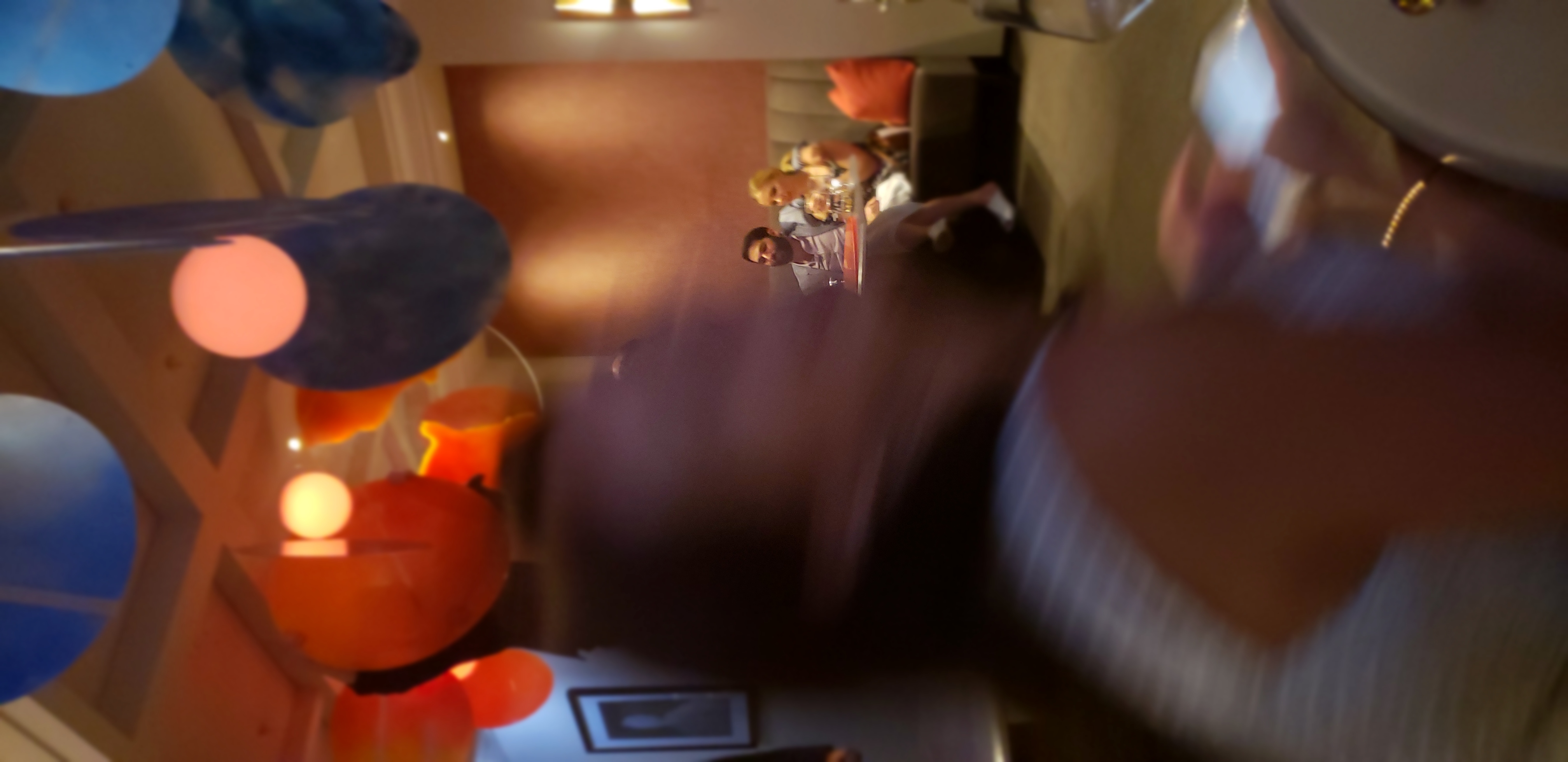The image depicts an extremely blurry view of a woman with long brown hair, seemingly in motion, making it difficult to discern the details of her facial features, though it appears she might be smiling. She is dressed in a sleeveless striped top with shades of light gray, white, and blue, and is holding a smartphone. In front of her, there is a light from the screen of her phone. She's positioned such that you see her profile and part of her back, suggesting she might be seated in a chair or couch in a living room setting. In the clearer background, there is a gray-scale padded booth or couch adorned with an orange throw pillow. Seated closely together at this booth is a couple; the woman has blonde hair and the man has black hair. They appear to be in an intimate pose, with the man possibly having his arm around the woman. The wall behind them has an orangey hue as if highlighted by the ambient light. Overhead, there are colorful lights featuring shades of blue, black, and two tones of orange, contributing to a warm and cozy atmosphere, though still indistinct due to the image's overall blur.